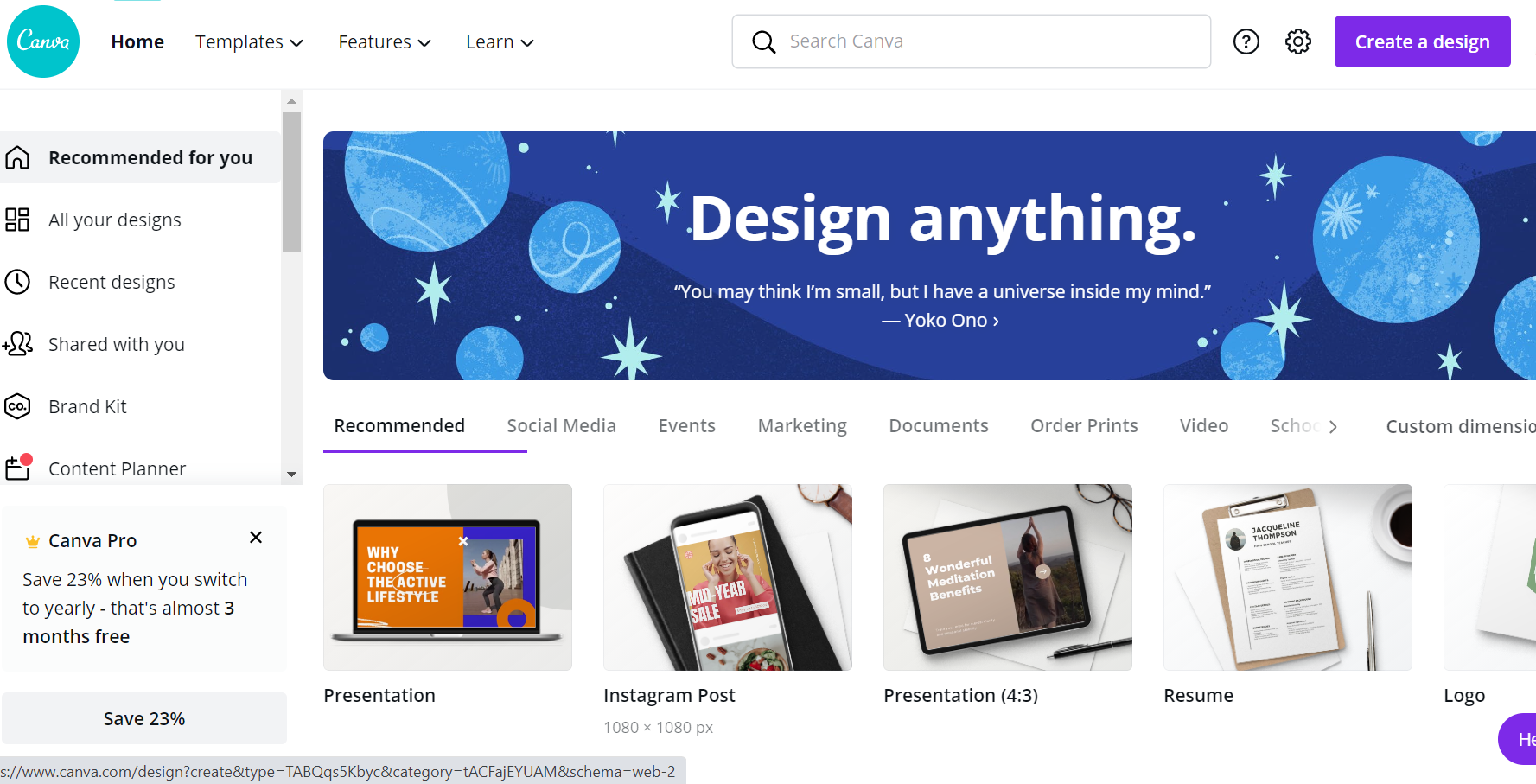The image depicts a screenshot of the Canva homepage. At the top left corner, a logo reading "CAMRA" (formatted as C-A-M-R-A) is displayed within a blue circle, written in script font. Along the top navigation bar, there are tabs labeled "Home," "Templates" with a drop-down arrow, "Features" with a drop-down arrow, and "Learn" with a drop-down arrow. A search bar labeled "Search Canva" with a magnifying glass icon is situated next to a question mark icon and a gear icon for settings. The "Create a Design" button is prominently displayed.

On the left sidebar, the following options are listed: "Recommended for You," "All Your Designs," "Recent Designs," "Shared with You," "Brand Kit," and "Content Planner." Below these, there is an advertisement for "Canva Pro," offering a 23% discount when switching to a yearly plan, equating to almost three months free, with a clickable button to save 23%.

The top of the webpage features a blue banner adorned with light blue planets and stars on a dark blue background. The banner includes a motivational quote from Yoko Ono: "Design Anything. You may think it's small, but I have a universe inside my mind."

Beneath this banner, there are five clickable buttons for different design templates: 
1. "Presentation" with a subtitle "Why choose the active lifestyle?"
2. "Instagram Post" with dimensions 180 by 180 pixels.
3. "Presentation" in a 4:3 ratio.
4. "Resume," accompanied by an icon depicting a resume on a table with a coffee cup.
5. "Logo."